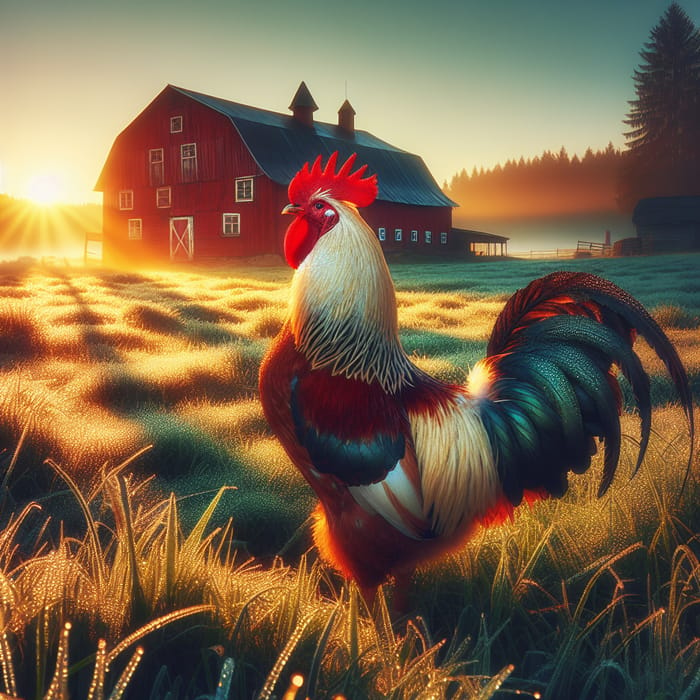A highly detailed digital artwork, possibly AI-generated or created with advanced 3D techniques, depicts an early morning scene on a farm. The central focus is a rooster with striking features: vibrant red wattles and comb, a brown body adorned with rich brown feathers, and a head covered in pristine white feathers. The early sunlight, just starting to rise above the tree line, casts a golden hue over the scene, illuminating the fine droplets of mildew on the grass, which glisten like tiny jewels. In the background, a robust red barn stands prominently, surrounded by a border of tall trees. The composition captures the serene beauty and crisp freshness of a morning in farmland, with the rooster exuding natural majesty amidst the tranquil setting.